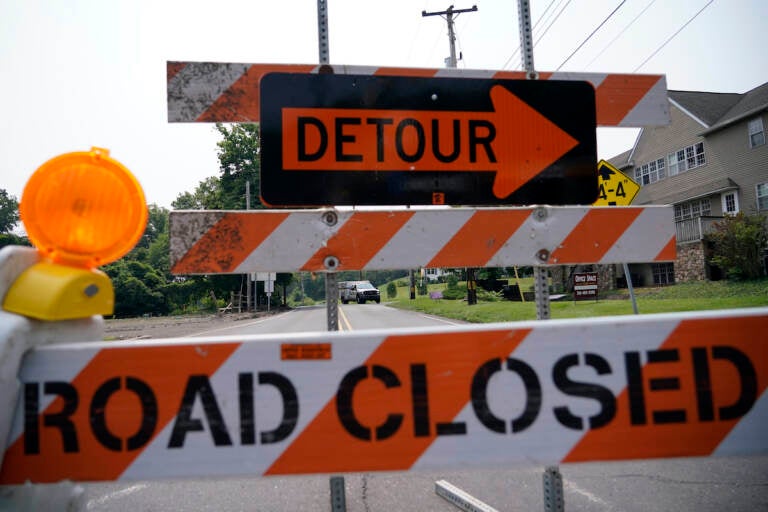The photograph, taken outdoors during the daytime, prominently features a construction sign centered in the frame. This sign is composed of three components: an upper section with an orange arrow pointing to the right and the word "Detour" on a black background, a middle section with diagonal orange and white stripes, and a lower section indicating "Road Closed" in black letters. The orange and white stripes accentuate the sign, and there is also an orange warning light positioned on its left side, which can flash. The sign is positioned directly in front of the camera, dominating the image and partially obscuring the background.

In the background, a road stretches out lined with grass and trees on either side. Visible in the distance are a couple of two-story houses, including a notable brown house, situated to the right. Further down the road, approximately half a mile away, there is a utility truck, but no specific details or lettering can be discerned on the vehicle. Additionally, there is a business sign in front of a building which remains illegible due to its small letters. Overall, the focus remains sharply on the "Detour Road Closed" sign, making it difficult to see much beyond it.